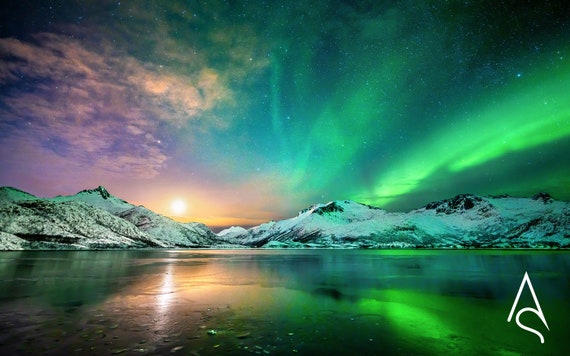This stunning photograph, reminiscent of a feature in National Geographic, captures the breathtaking display of the Northern Lights over an Arctic landscape. On the left side, vivid green auroras light up the night sky, gradually transitioning to pink and orange hues on the right, indicative of a sun partially hidden behind the horizon. The mountains, blanketed in pristine snow, stand majestically in the background, while a serene body of water occupies the foreground. The water's surface mirrors the vibrant celestial light, with shades of deeper green, purple, and teal reflecting vividly. Also noticeable is a graphic symbol in the bottom right corner, outlined in white, possibly signifying a tourism logo or the photographer's signature. The entire scene is captured in exquisite color, making it a visually captivating piece.